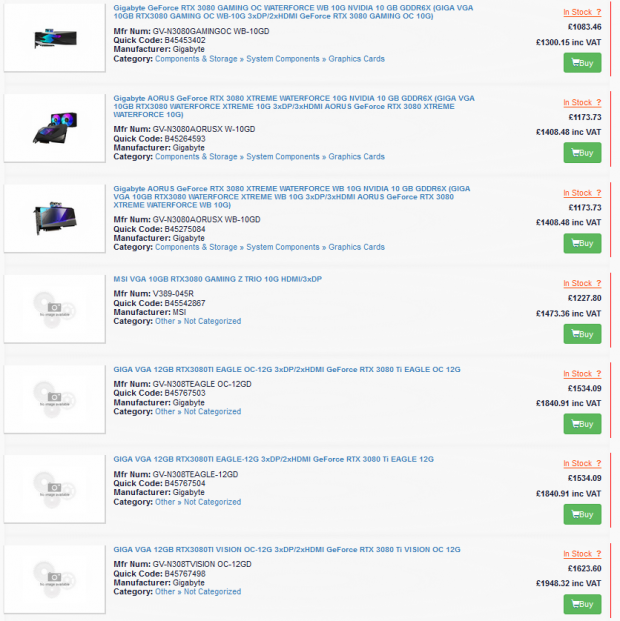Screenshot from an online shopping website showcases a series of listings primarily for graphics cards or other gaming-related hardware. The first three listings are categorized under "Components & Storage" and "System Components - Graphics Cards," while the remaining four are labeled as "Other" and are not categorized. 

Each listing features a blue product name and is accompanied by a manufacturer number, quick code, manufacturer details, and category. The top three items display images of the graphics cards, each with a distinct color scheme incorporating black, purple, and teal. In contrast, the bottom four listings only show a generic placeholder image of a white square with gray circles and a camera icon.

Marked with orange "In Stock" notifications, all items are priced in black text, along with a "Price With VAT" detail. A green shopping cart icon with a white "Buy" label is present next to each listing. Additionally, a red line appears next to the "Buy" button. The font used is clear and easy to read, despite the repetitive and lengthy nature of the names and codes.